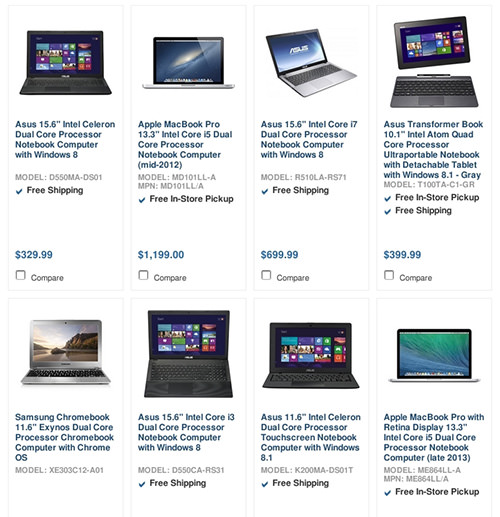The screenshot captures the search results for laptops, displaying a variety of options across different brands and specifications. It features four visible laptops, ranging in price from $329 to $1,211.99. The laptops listed are from brands such as Asus, Apple, and Samsung, spanning multiple configurations.

From left to right, the top row includes:
1. An Asus laptop with a 15.6-inch display and Intel Celeron processor.
2. An Apple MacBook Pro featuring a 13.3-inch display.
3. Another Asus 15.6-inch laptop, this one with an Intel Core processor.
4. An Asus Transformer Book, which features a detachable screen, allowing it to function similarly to an iPad.

In the bottom section, additional laptops are visible:
1. A Samsung Chromebook with an 11.6-inch display.
2. Another Asus 15.6-inch laptop.
3. An Asus with an 11.6-inch display.
4. Another Apple MacBook Pro with a 13.3-inch display and Intel Core processor.

Out of these options, seven of the laptops offer free shipping, with the exception of the Samsung Chromebook. This variety of laptops is likely the result of someone searching online for the ideal laptop purchase.